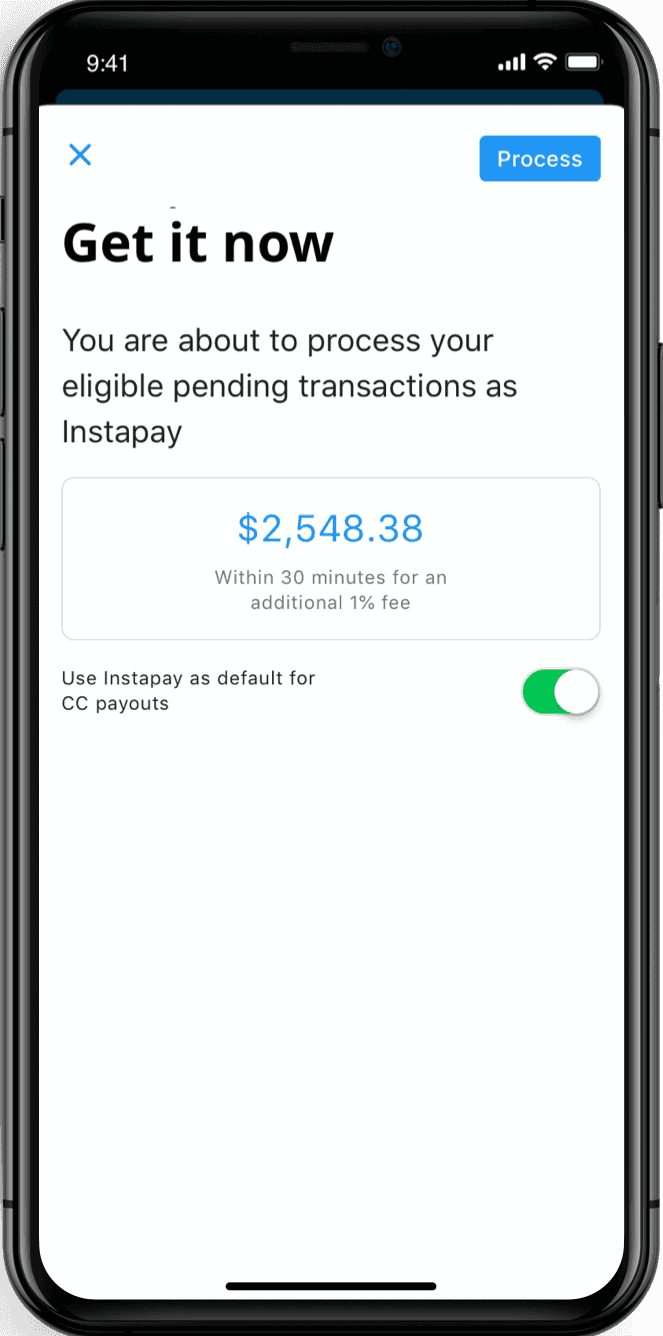The image showcases a black smartphone displaying a website interface. At the top right of the screen, the battery icon is fully charged, next to a fully powered Wi-Fi symbol and a phone signal strength at four bars. The top left corner shows the current time as 9:41. 

In the middle of the screen's header, the phrase "Get it now" is written in black text. The top left features a blue "X" icon, while the top right hosts a rectangular border with the word "Process" inscribed inside. 

The central section of the display contains a notification reading, "You are about to process your eligible pending transactions as Instapay." Beneath this message, a box highlights the amount "$2548.38" to be processed within 30 minutes for an additional 1% fee. Below, the notification offers an option with the text, "Use Instapay as default for CC payouts," accompanied by a small empty space to the right, ending with a green checkmark.